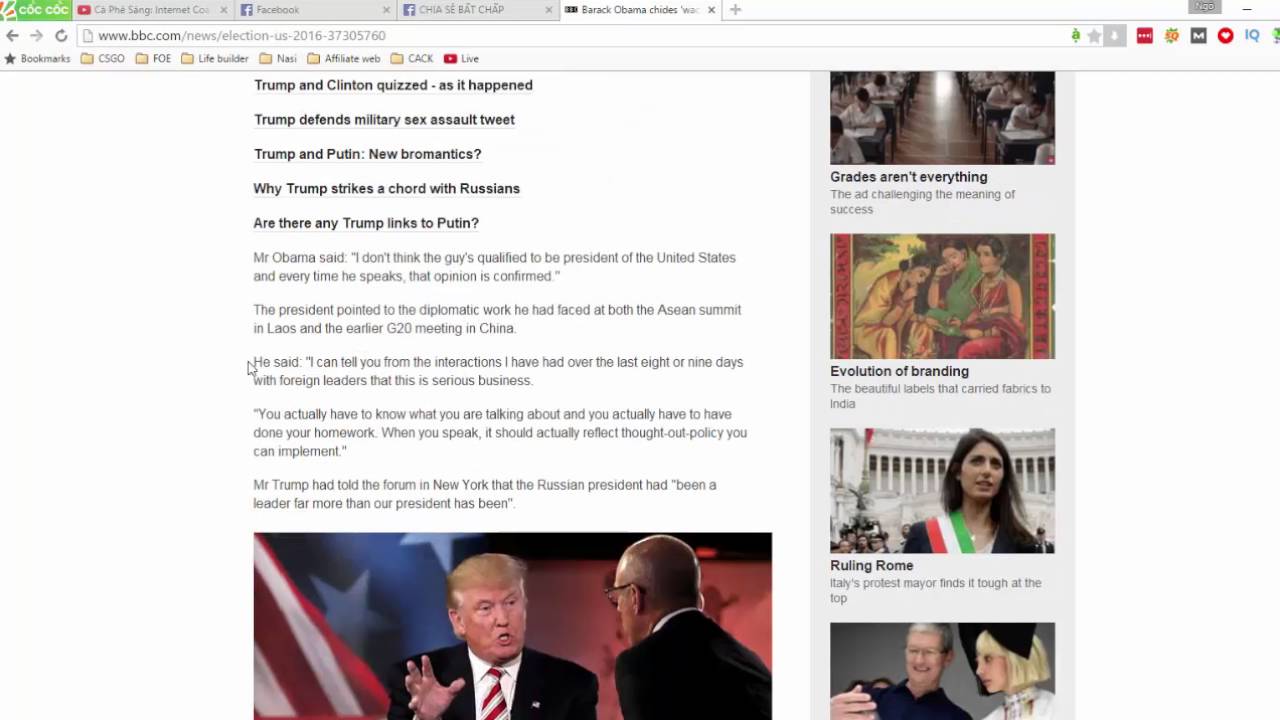Screenshot from a BBC News article dated 2016, as indicated by the web address bar. The webpage is part of the "BBC.com/news/elections/us/2016" segment, featuring an image of Donald Trump engaged in a conversation with a bald, bespectacled gentleman. An American flag is visible in the background, suggesting a patriotic or political setting. The article headline and subheadings discuss various topics including Trump's defense of a military sex assault tweet, his relationship with Vladimir Putin referred to as "bromantics," and the potential connections between Trump and Putin. There's a bold statement from then-President Obama questioning Trump's qualifications for the presidency. Obama, speaking at an ASEAN summit in Laos and a G20 meeting in China, emphasized the importance of knowledgeable and thoughtful diplomacy. In a sharp contrast, Trump praised the Russian president as a more effective leader than Obama during a forum in New York. The webpage also contains side articles on topics such as the insignificance of grades, the evolution of branding, and historical insights on ruling Rome. The browser toolbar shows several bookmarks and tabs, including a Facebook page and a site in a foreign language labeled "Qi Sao Bot Chop" and "CBC COC."